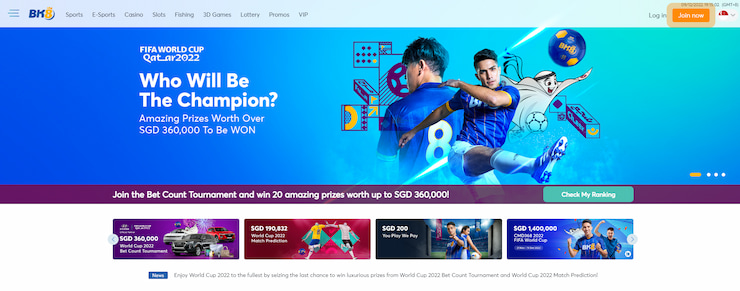Here is a cleaned-up and detailed caption for the described image:

---

**FIFA World Cup 2022 in Qatar: Who Will Be the Champion?**

Join the excitement and seize the chance to win 20 amazing prizes worth over SGD 360,000. Participate in the "Bet, Count, Tournament and Win" for a shot at luxurious rewards. The enticing green "Check My Ranking" button adds to the thrill, all set on a striking purple strip.

The vibrant image showcases two soccer players in blue uniforms, energetically competing on a blue field. Their dynamic movements and pleated shoes are vividly depicted as they chase the soccer ball. Among them, a ghostly figure adds an intriguing twist to the scene. 

Highlighted prizes include:
- Automobiles from the World Cup 2022 Red Court Tournament
- Participation worth SGD 190,000 in a World Cup 2022 match
- A special reward with the motto "You Play, We Pay" valued at over SGD 200,000

Don't miss out on the ultimate World Cup 2022 experience. Enter now to maximize your chances of winning luxurious prizes through the Bet Court Tournament and Match Prediction events. 

---

Feel the thrill of the FIFA World Cup 2022 and make your predictions now!